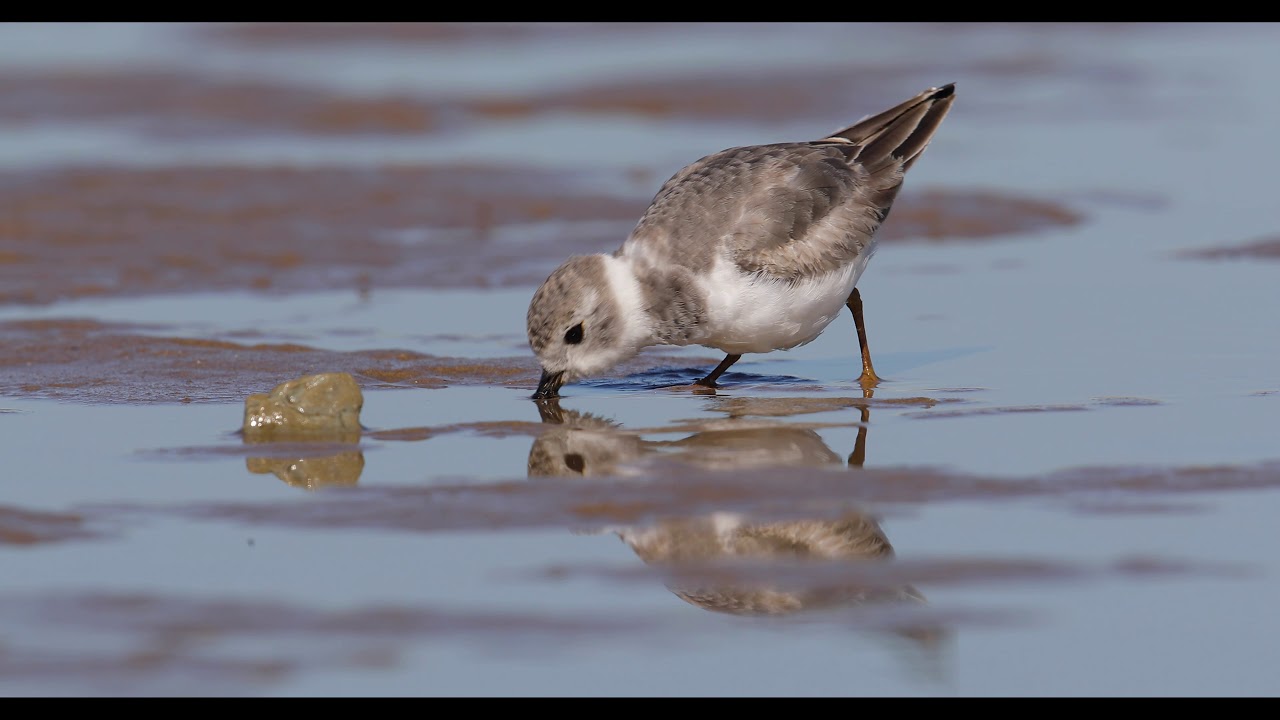In this photograph, we see a small bird, potentially a duck or a sparrow-like bird, standing in very shallow water. The bird’s body is predominantly gray with a white chest and a white ring around its neck. Its tail feathers are darker gray, almost black, and it has a beady black eye. The bird is captured mid-action, dipping its black beak into the water, and both its reflection and that of its surroundings can be seen in the photo.

The water itself is primarily blue with a brown texture on top and splotches of dark brown scattered throughout, indicating the shallow depth. There are visible patches where the water is so shallow that dirt or wet sand is exposed. In front of the bird, there is a small wet rock protruding from the water. Additionally, there appears to be a piece of a bottle with brown dirt on it located in the water near the bird. The reflection of the bird is visible at the bottom part of the image but is partially obscured by ripples in the water. The overall scene is calm, with the bird's reflection adding a serene quality to the image.